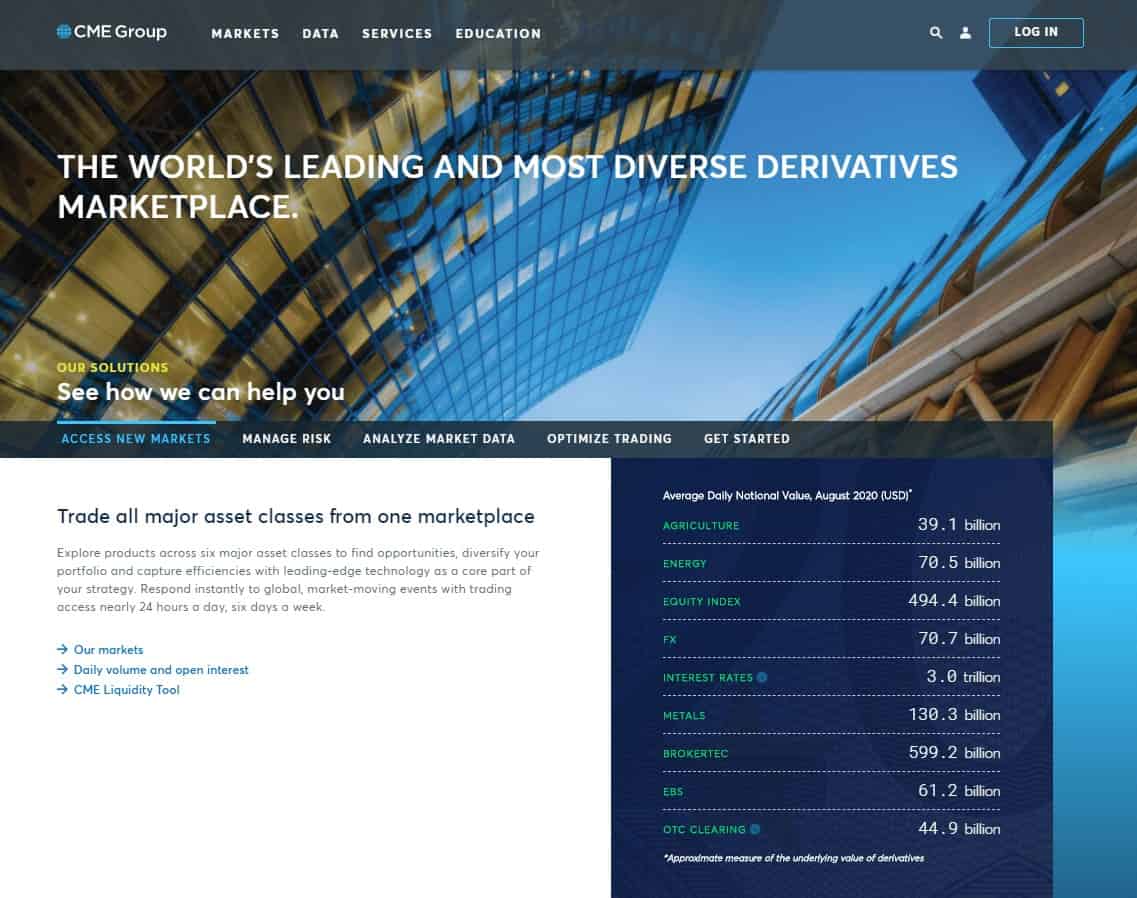This screenshot features the homepage of the CME Group website, tailored for desktop viewing. The main image spans wider than it is tall, displaying a semi-transparent upper banner in dark navy blue fading into near black. In the upper left, the CME Group logo—a blue circular emblem—is prominently placed alongside the company name in white text. Adjacent to the logo are menu tabs labeled "Markets," "Data," "Services," and "Education," also in white font. On the opposing corner, a "Login" button is situated for user access.

The background image provides a dramatic upward view from ground level of towering skyscrapers against a clear blue sky. Overlaid on this backdrop in large white font are the words, "The World's Leading and Most Diverse Derivatives Marketplace," with the phrase "Our Solutions" highlighted in yellow beneath it, followed by "See how we can help you" in white font.

Below this, navigation tabs offer various site sections, with "Access New Markets" currently selected. In the lower left corner, a white box contains text promoting the site's capabilities: "Trade all major asset classes from one marketplace," alongside some additional text and hyperlinks for more detailed information. The lower right corner features a blue square displaying diverse market statistics related to average daily national values in categories such as agriculture, energy, equity index, and foreign exchange (FX), emphasizing the site's focus on derivatives marketplace trading.